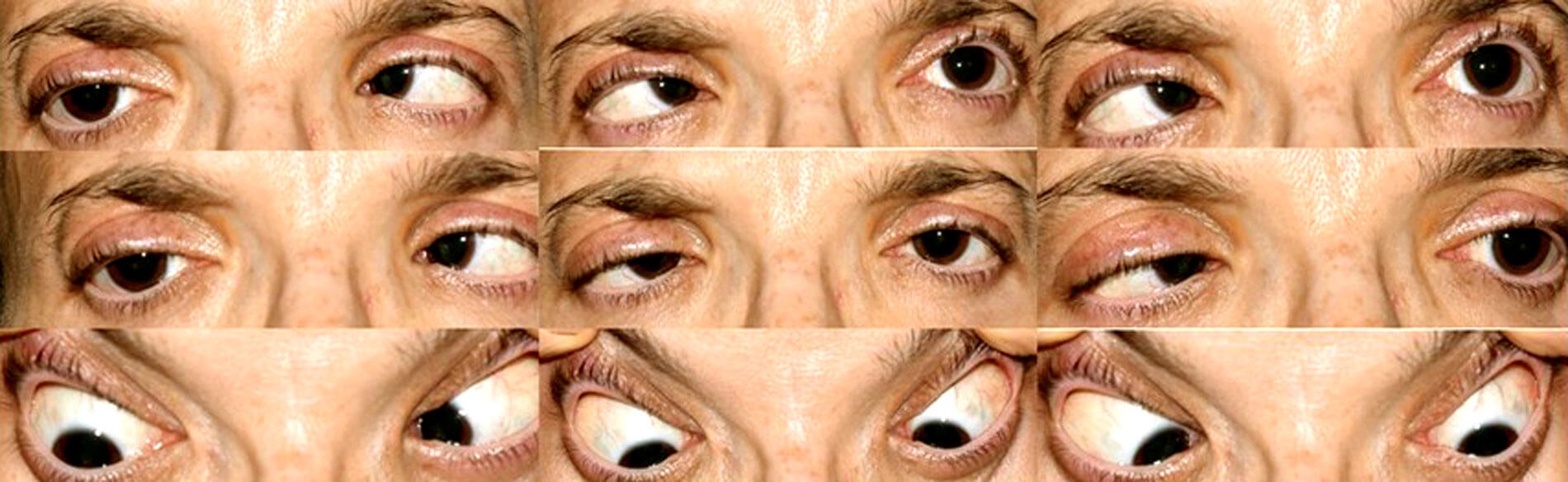The image features a close-up compilation of nine pictures of what appears to be the same pair of dark brown eyes, arranged in a grid with three rows and three columns. The photos only capture the eyes, the top of the nose, part of the eyebrows, and a bit of the forehead, with the rest of the face not visible. The different eye positions in each photo give off a somewhat eerie and strange vibe. 

In the top row, the left eye in the first picture looks forward while the right eye appears crossed. In the second and third pictures of the top row, the eye positions are reversed, with the right eye looking forward and the left eye crossed towards the nose. The second row mirrors this sequence with again varying positions of the eyes crossing and looking forward. 

The bottom row displays the eyes in a more surprised or exaggerated expression, with the eyelids pulled back farther than normal, making the whites of the eyes much more pronounced. In this row, the eyes are predominantly looking downward. The face belongs to a middle-aged person with olive-tan skin and black eyebrows, but there are no further identifying details or contextual information provided.